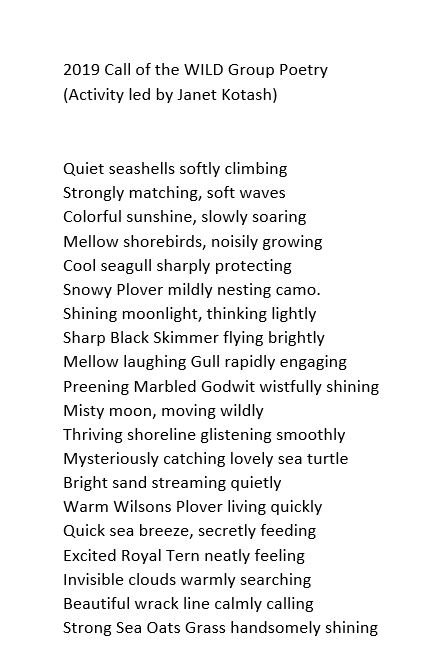The image displays a poem printed in about 8-point black font on a white background, titled "2019 Call of the Wild Group Poetry" with the note "activity led by Janet Kotash." The poem reads:

    Quiet seashells softly climbing,
    Strongly matching soft waves,
    Colorful sunshine slowly soaring,
    Mellow shorebirds noisily growing,
    Cool seagulls sharply protecting,
    Snowy plover mildly nesting camo,
    Shining moonlight thinking lightly,
    Sharp black skimmer flying brightly,
    Mellow laughing gull rapidly engaging,
    Preening marbled godwit wistfully shining,
    Misty moon moving wildly,
    Thriving shoreline glistening smoothly,
    Mysteriously catching lovely sea turtles,
    Bright sand streaming quietly,
    Warm Wilson's plover living quickly,
    Quick sea breeze secretly feeding,
    Excited royal tern neatly feeling,
    Invisible clouds warmly searching,
    Beautiful wrack line calmly calling,
    Strong sea oats grass handsomely shining.

The poem appears to have been created as a group activity under the guidance of Janet Kotash. The descriptive verses evoke imagery of a serene, thriving shoreline with various birds, sea creatures, and natural elements interacting harmoniously.